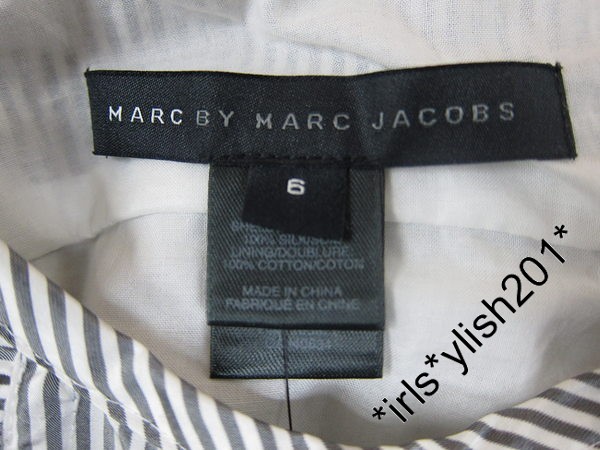This photograph provides a close-up view of a clothing label from a shirt designed by Marc by Marc Jacobs. The image focuses primarily on the label, a narrow black rectangle bearing the brand name "MARK" in white and "BY MARK JACOBS" in gray. Below the main label, there are three additional black tags: one indicating the size ('6' in white on a gray background), another detailing the fabric (100% cotton) and manufacturing origin (made in China), and a third, more obscure tag. A string attaches the price tag to these labels, but the price itself is not visible. The fabric of the shirt is notably striped in gray and white on the exterior, with a solid white interior. An inscription on the image itself reads "*IRLS*YLISH 201*."